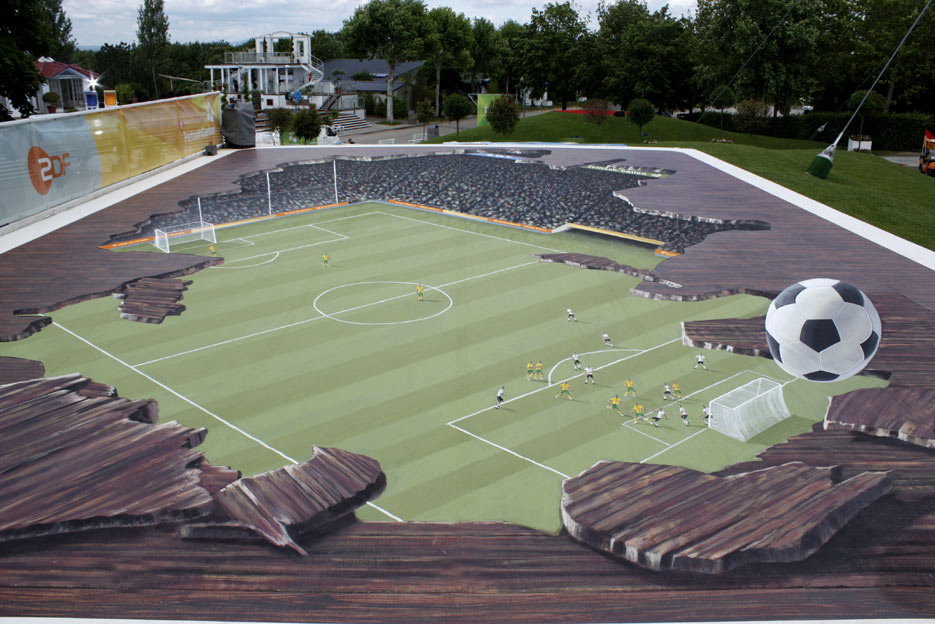This photograph depicts an outdoor 3D mural on a brick courtyard, illustrating a vividly detailed soccer match. The expertly crafted mural creates the illusion of a soccer stadium, with one team dressed in yellow and green and the other in black and white. The yellow team is on the offensive, visible through dynamic positions on both sides of the pitch, with the black-clad team defending a small white net. The 3D effect is enhanced by depicted wooden fragments seemingly breaking away to reveal a crowd of indistinct spectators engrossed in the game. 

Adjacent to the mural, on the left, is a wall that appears to be made of paper, adorned with a red circle containing the number "2," and the letters "D" and "F" in red text on a gray background. Accompanying this is a large yellow triangle, an orange trapezoid with white text, and another yellow triangle. 

The scene is set on an overcast day with a light blue sky, scattered with clouds. Behind the mural wall, a white house with a maroon roof sits, its entrance flanked by dark blue and orange chairs made with white wood. Extending from left to right, a tree line frames the background, complemented by fresh green grass with three small plants or trees at its center. The right side of the photo captures the edge of a gray road and a dark green cylindrical object connected to an upward wire. There is also a larger building under construction next to the paper wall, featuring a white facade and a gray roof with large cobblestones descending downward.

Overall, the photo masterfully combines the elements of the mural and its surroundings to create a richly detailed and engaging image.